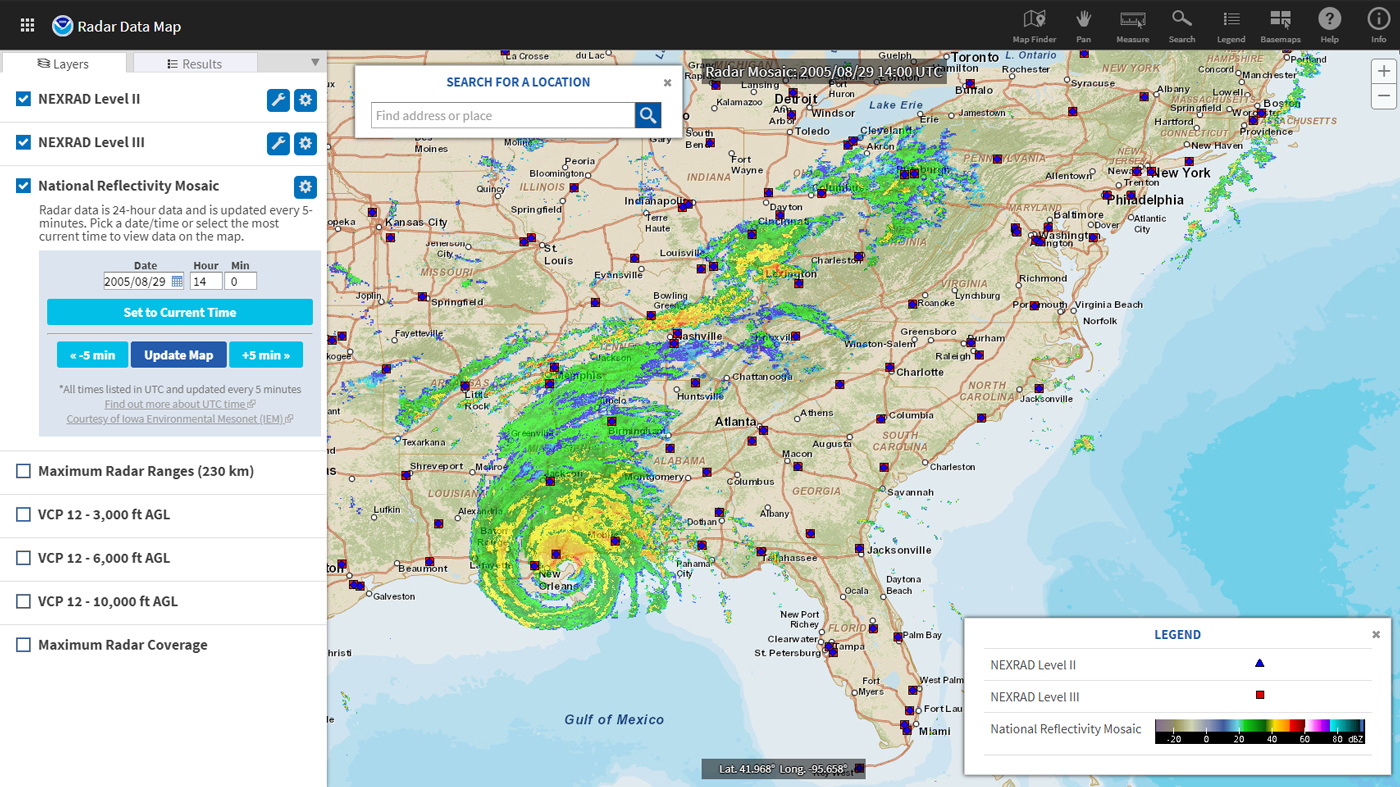This is an image of a weather radar data map screenshot from a weather viewing website. At the top of the image, a black bar prominently displays the title "Radar Data Map." To the left, a vertical column lists selected radar data layers: NEXRAD Level 2 and NEXRAD Level 3 with corresponding blue checkmarks, a wrench icon, and a gear icon indicating settings options. Below them, the National Reflectivity Mosaic is also selected, marked by another blue checkmark and gear icon.

The main section of the image shows a detailed map of the United States, spanning from Texas to the East Coast, including the Gulf of Mexico, Georgia, Florida, and all the way up to New York. The map highlights a significant weather event—a hurricane or large storm—centered over Louisiana, depicted with a mixture of green, yellow, orange, and blue colors. The storm's reach extends from the Gulf of Mexico up to Lake Erie and the upper corner of Virginia, indicating its extensive trail across the country. Additionally, the ocean surrounding the U.S. is visible, further framing the impact of this substantial weather system.